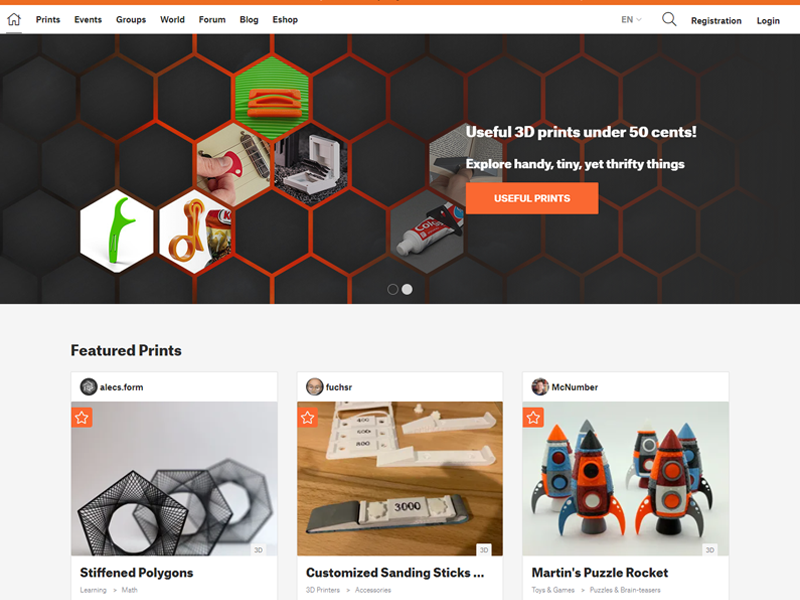This is a detailed screenshot of a webpage dedicated to affordable 3D printing. The top section showcases a striking black background adorned with a red honeycomb pattern. Each honeycomb cell contains a unique photograph, including images of a toothpaste tube, a bottle opener, a dental floss holder, and a guitar pick, among other unrelated small items. Overlaid on this honeycomb banner are the bold words, "Useful 3D Prints Under $0.50," highlighting the budget-friendly nature of the prints. Below this, a subheading reads, "Explore handy, tiny, yet thrifty things," inviting users to discover these economically priced items. An attention-grabbing orange button labeled, "Useful Prints," stands out, ready to guide users to more detailed content.

Beneath this introductory section, there is a featured prints bar displaying several intriguing 3D print options. The first image features a "3-polygon" design, the second image depicts “sending sticks,” which resemble small feet typically used under a box fan. The third image displays "Martin's puzzle rocket," showing colorful, buildable rocket pieces likely intended for children to assemble.